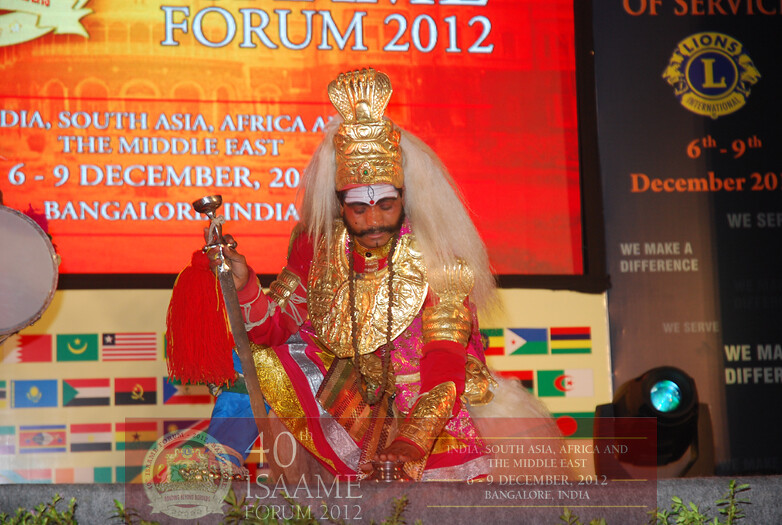A gentleman of East Indian descent is adorned in elaborate traditional attire, featuring a highly ornamental gold headdress with cascading feathers or tulle, and a white scarf beneath. His prominent and decorative mustache extends to his ears, adding to the regal appearance. He wears an intricately designed gold breastplate necklace, along with gold-embellished sleeves reminiscent of military attire over a red tunic, and a heavily ornamented belt. In his right hand, he holds what appears to be a scepter. 

Behind him, a bright yellow and red banner displays "Forum 2012" in white letters, with the text "India, South Asia, Africa, and the Middle East, 6 to 9 December 2012, Bangalore, India." An off-white banner below showcases many flags. Additionally, a deep black setting houses a blue jewel on the left. A brown banner marked with an "L" indicates the Lions Club, accompanied by their slogan, "We make a difference." The words "of service" are above the Lions logo. At the bottom, the inscription "40th Ismail Forum 2012" appears next to an insignia, with additional data to the right. The entire scene is vibrant and colorful, resonating with cultural significance and celebration.